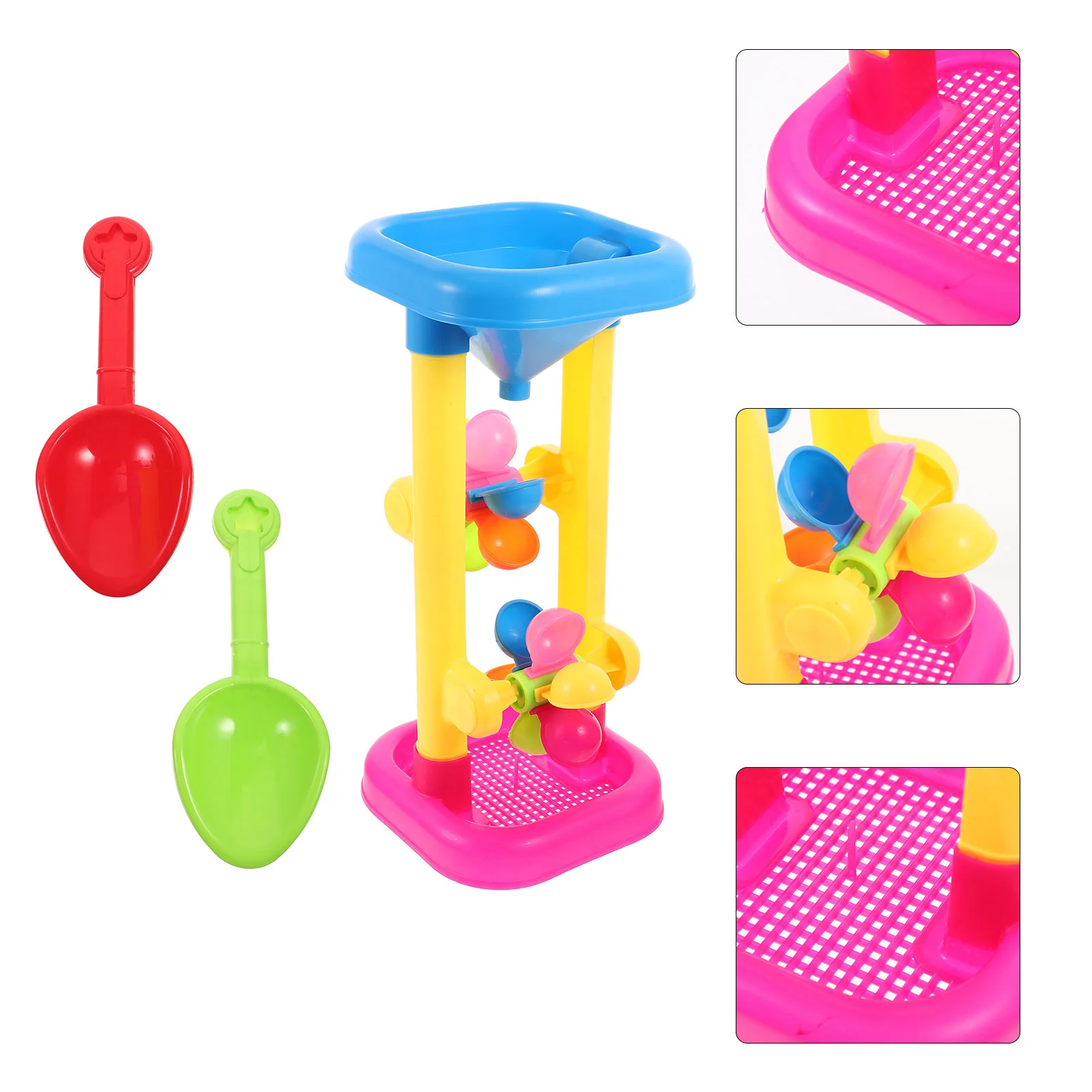The image depicts a colorful children's beach playset designed like a miniature Rube Goldberg machine. The toy features a blue square funnel at the top, leading to two vertical spinning windmill structures adorned with cups or scoops in vibrant colors—blue, pink, yellow, fuchsia, and green. These spinning components are positioned on a frame with a pink base, which has holes for sand drainage. The windmill-like scoops are arranged to spin and allow sand to flow through them, showcasing a kinetic display when in use. To the side of the main contraption, there are two small shovel-like scoops—one red and one neon green—each with a star design on the handle. These additional tools are intended for handling the sand that powers the spinning mechanism. The entire assembly is set against a white background, with close-up views of the pink base and the spinning cup structures highlighting the toy's details.